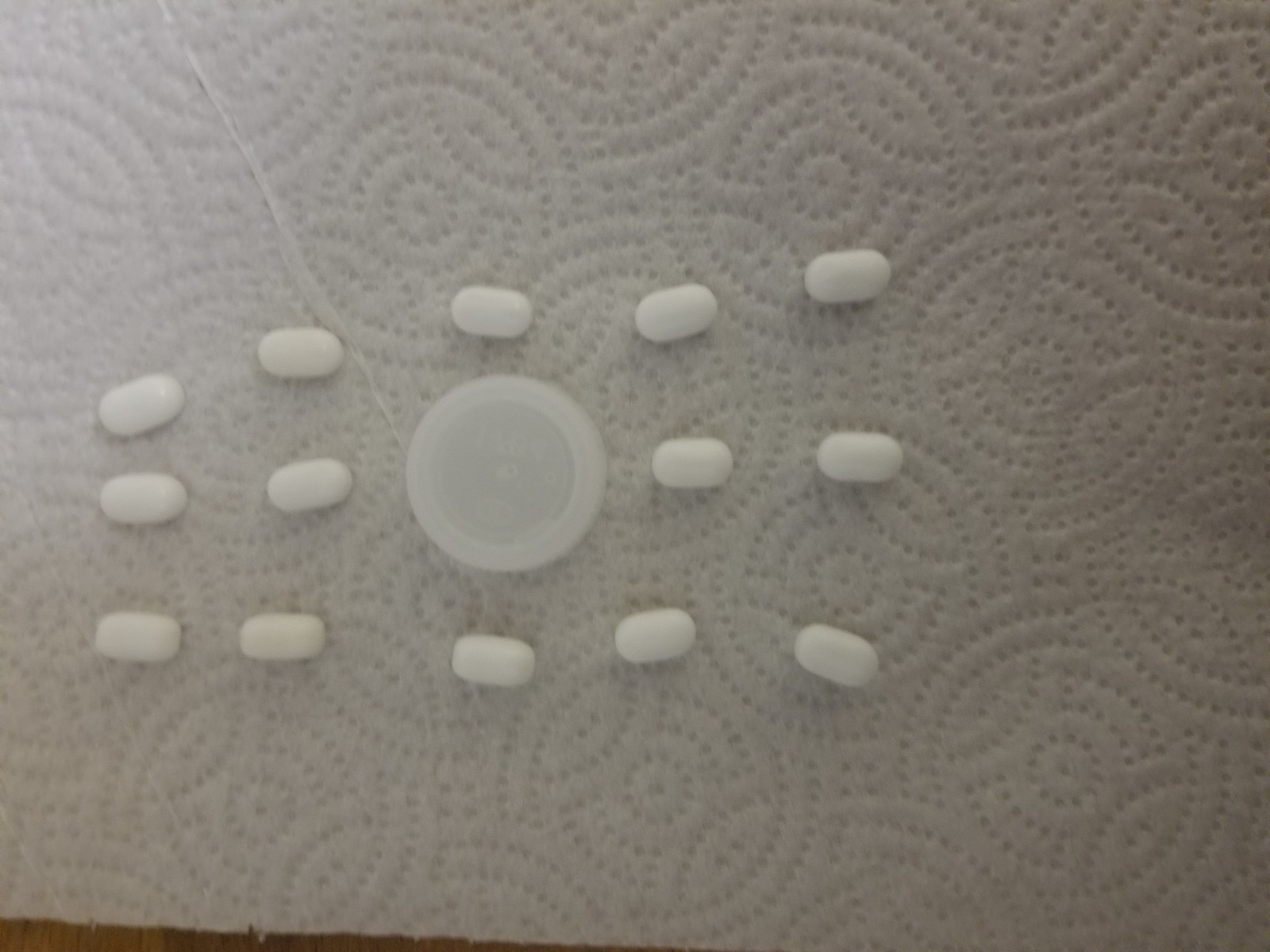This image shows a white paper towel with a circular embossed design in the background. On top of the paper towel, there are 14 slightly shiny, oblong, cylindrical pills arranged in three horizontal rows. The top row has five pills, the middle row has four pills with a round translucent plastic medicine bottle cap in the center, and the bottom row has five pills, all spaced about an inch apart. The overall arrangement is slightly fanned out towards the right side. The translucent cap in the middle row has a slightly darker area around its rim.